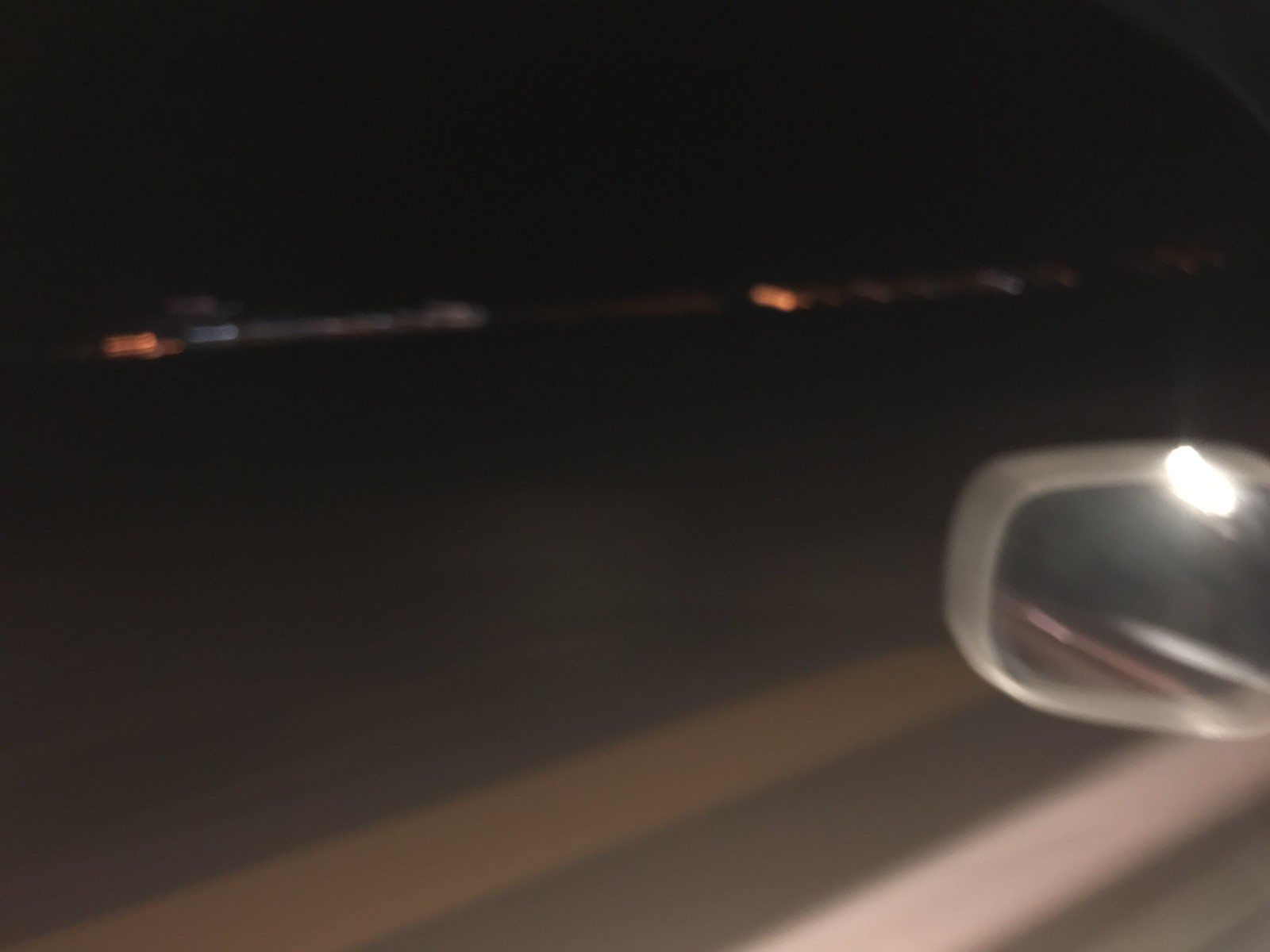This image appears to be captured from within the passenger compartment of a moving vehicle, specifically from the perspective of the front left seat. Prominently featured in the shot is the rearview mirror on the driver's side, which has a white housing. The mirror reflects a concentrated flash of light, likely from the camera capturing the image, evident both on the mirror's glass and housing. To the immediate left outside of the vehicle, one can observe a solid white line, and further left of that, a solid yellow line, indicating lane markings on a roadway. The road surface appears dark and flat, extending towards a horizon. In the distance, there are orange and white lights shining from a short building, possibly a warehouse, characterized by its single-story height. Beyond this structure, the backdrop is uniformly black, suggesting it is nighttime with no additional sources of light visible beyond the warehouse building.